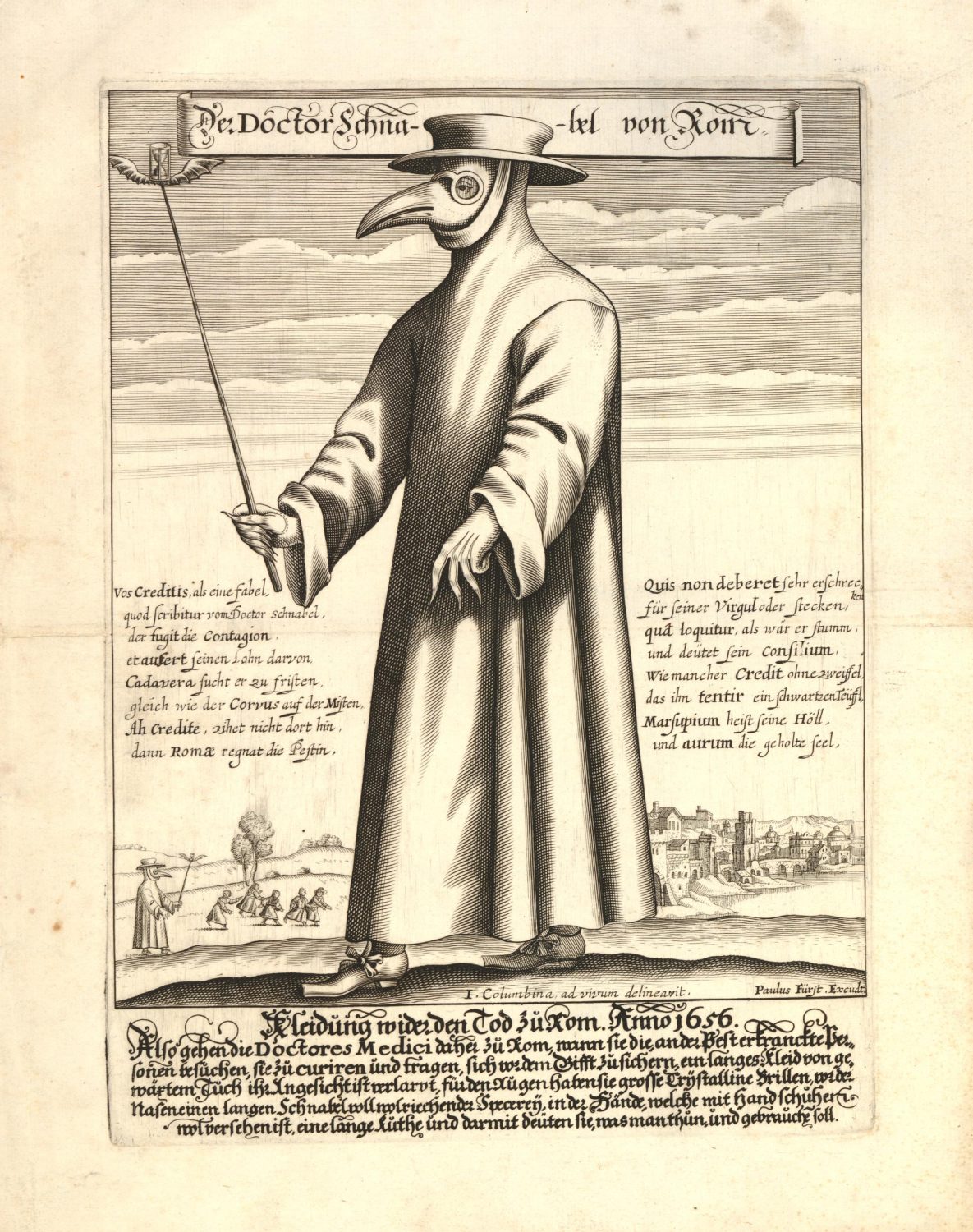The image depicts an eerie, historical drawing on a yellowed, creased, and spotted piece of paper, possibly an etching or computer-generated illustration reminiscent of aged parchment. The central figure is titled "Dr. Schnabel von Gorm" at the top of the image, rendered in a blend of brown and black ink. This character is garbed in a voluminous, flowing robe that drapes from beneath a short top hat down to its pilgrim-like shoes, which are adorned with small ribbons at the ends. The figure's face is peculiar, resembling a bird's head—perhaps a gull or a penguin—with a beak that appears to be part of its actual face. This unsettling visage is complemented by glasses over its eyes.

The figure clutches a staff, topped with an hourglass and winged embellishment, enhancing its eerie presence. Surrounding the main figure are intricate calligraphic writings in an unreadable language, adding an air of mystery. The backdrop showcases a pastoral village scene with rolling hills, a tree, and clouds in the sky. There are smaller figures, possibly farmers, wielding similar staffs or rakes, and people or children fleeing towards the village. The bottom of the image features additional unreadable calligraphic writing, further contributing to the enigmatic atmosphere of the illustration.